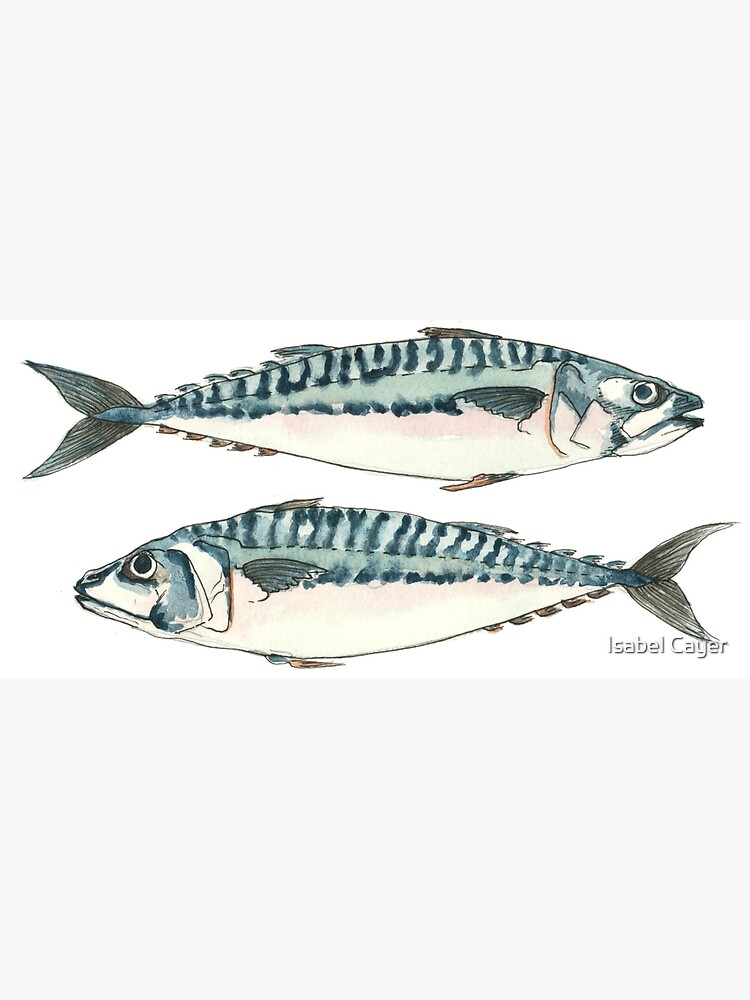This art print features a detailed and stylistic depiction of a tuna fish from two different perspectives: the left-facing profile is positioned at the bottom while the right-facing profile is at the top. The fish appears within a thin, white rectangular space, flanked by larger light-gray rectangles on the top and bottom. Each illustration showcases the same fish rendered with watercolors, accentuating its sleek and cylindrical form. The fish displays a white underbelly with a hint of beige, while its midsection is marked by a light pink stripe. The upper body transitions into varying shades of blue, capped by a teal stripe along the back with vertical, darker blue lines. The fins are primarily blue, and the tail is bifurcated with a light bluish hue. The fish's eyes have a hazy blue tint, featuring black pupils. Artist Isabelle Keyer's signature is present in white in the lower-right corner of the print.